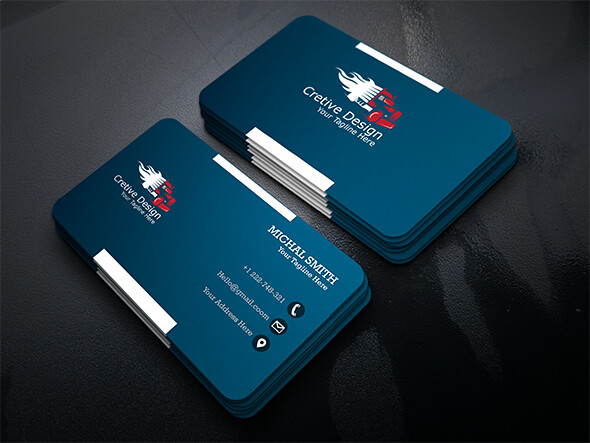The image showcases two stacks of business cards, predominantly navy blue in color, placed on what appears to be a brown and grey countertop with a slightly wet or dark leather-like background. One stack prominently displays the text "Creative Design" (misspelled as "C-R-E-T-I-V-E-D-E-S-I-G-N") in white letters, accompanied by a logo of a red truck with white flames on the blue background, and the tagline "Your tagline here." The other stack contains a sample card with "Michael Smith" written at the top, followed by "your tagline here," a phone number "+1-223-740-331," and an email address "hello@gmail.com." Additionally, it includes an emblem for the email and a placeholder text "your address here" along with a location emblem. The cards are roughly the size of credit cards but more closely resemble business cards based on the text and format. The light hits the table and cards, highlighting their sleek, professional design.